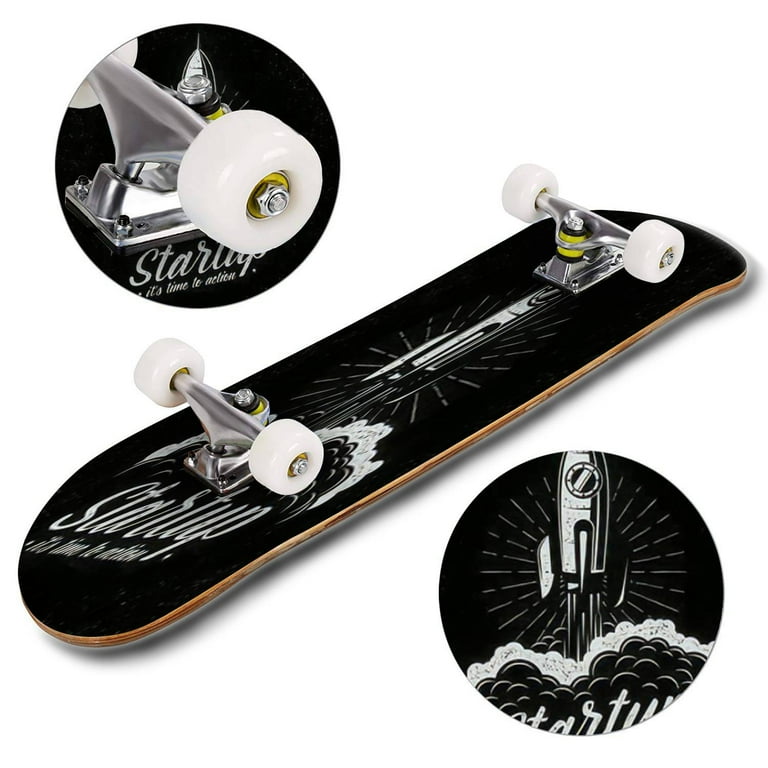This image features a skateboard displayed against a white background. The skateboard is flipped upside down, showcasing its underside. The underside of the skateboard is predominantly black, adorned with a white graphic design. The design includes an illustration of a rocket ship and the word 'Starship' written in cursive. The skateboard is equipped with white wheels. There are two circular close-up insets: one at the top left highlighting the white wheels, and another at the bottom right providing a detailed view of the rocket ship graphic. The metal parts of the skateboard are silver, and the edges have a hint of brown. The clean, minimalist presentation suggests it might be marketed for sale online.